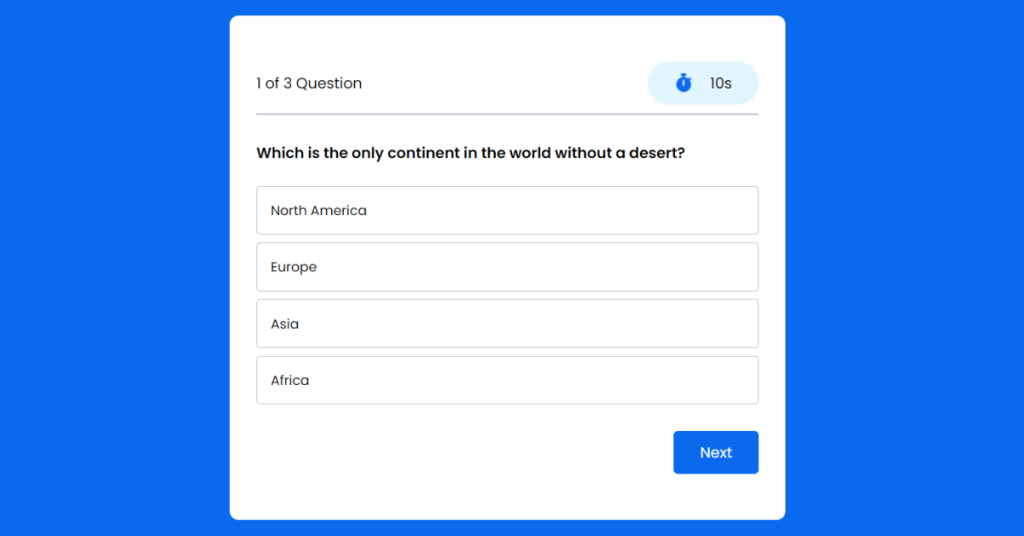The image features a simple blue background with a prominent white box at its center. Inside the white box, there is a multiple-choice quiz layout. In the top-left corner of the box, text indicates that this is "Question 1 of 3." To the right of this, a horizontal blue oval contains a timer set to "10s," followed by a gray line.

Beneath the timer, a bold, black question reads: "Which is the only continent in the world without a desert?" The question is followed by four answer options displayed in white boxes with gray borders. The options are:
1. North America
2. Europe
3. Asia
4. Africa

At the bottom-right corner of the white box, there is a blue "Next" button. The rest of the background remains a plain blue, adding to the simplicity of the design.